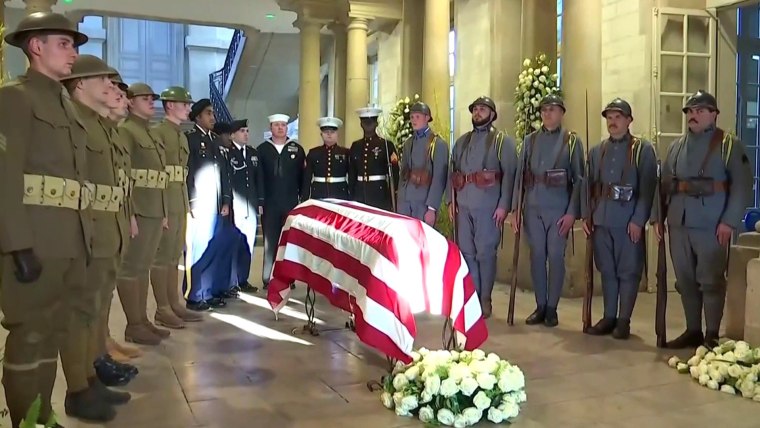The image depicts a solemn military funeral ceremony. In a U-shape formation, various servicemen stand at attention. On the left, approximately five British soldiers are dressed in brown uniforms and flat brown hats. Adjacent to them, about five American servicemen, including sailors, Marines, and Air Force personnel, are similarly lined up. To the right, a contingent of French soldiers in gray uniforms and metal helmets completes the formation. All troops exhibit a serious and proper demeanor.

At the center of the scene lies a casket draped with a red and white striped American flag, signifying that the deceased is American. A bouquet of white flowers rests at the foot of the coffin, and another cluster of white blooms lies on the floor near the French soldiers. The ceremony takes place in an ornamental building with yellow walls, decorative columns, and heavy wooden beams. On the right side of the image, there is a door with a glass pane, while another door is visible at the top of a staircase on the left. Sunlight streams through, illuminating the tan-tiled floor of this somber setting.